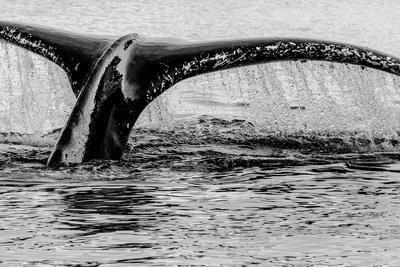This black-and-white photograph captures a dynamic close-up of an orca whale's tail fin, dramatically flipping out of a large body of water. The image is predominantly composed of various shades of black, white, and gray, emphasizing the contrast between the water and the whale's tail. The tail fin spans the entire width of the image, with its tips extending beyond the frame, and occupies the upper half of the scene. Water cascades off the tail, creating faint lines and splashes that disturb the otherwise calm surface. The lower part of the tail, partially submerged, is visible towards the bottom right, reflecting light suggesting a back-top light source. The image is devoid of any other elements or signatures, enhancing the focus on the orca whale's powerful movement.